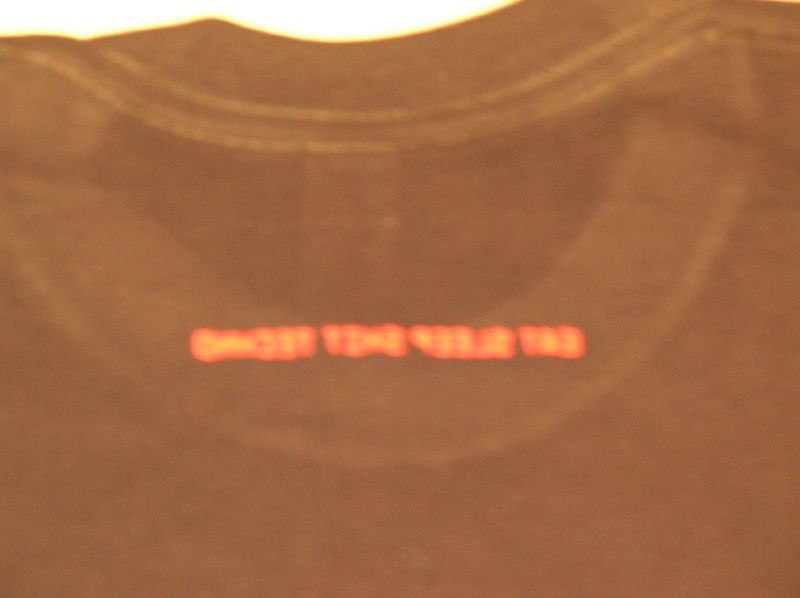The image is an extreme close-up photograph of a black t-shirt collar, likely from the back of the shirt given the shorter depth of the collar. The t-shirt appears to be laid flat for the picture. The focus is on a section where blurred and distorted red or orange text runs across the fabric, making it difficult to discern the content. The blurred text seemingly consists of four words or sets of characters, giving it a slightly chaotic appearance reminiscent of an inversion or mirrored effect. The background above the collar is white, with part of a hang tag visible, suggesting it might have been partially ripped off. The overall impression is one of simplicity and ambiguity, with the blurry text and minimalist setting creating a sense of mystery.